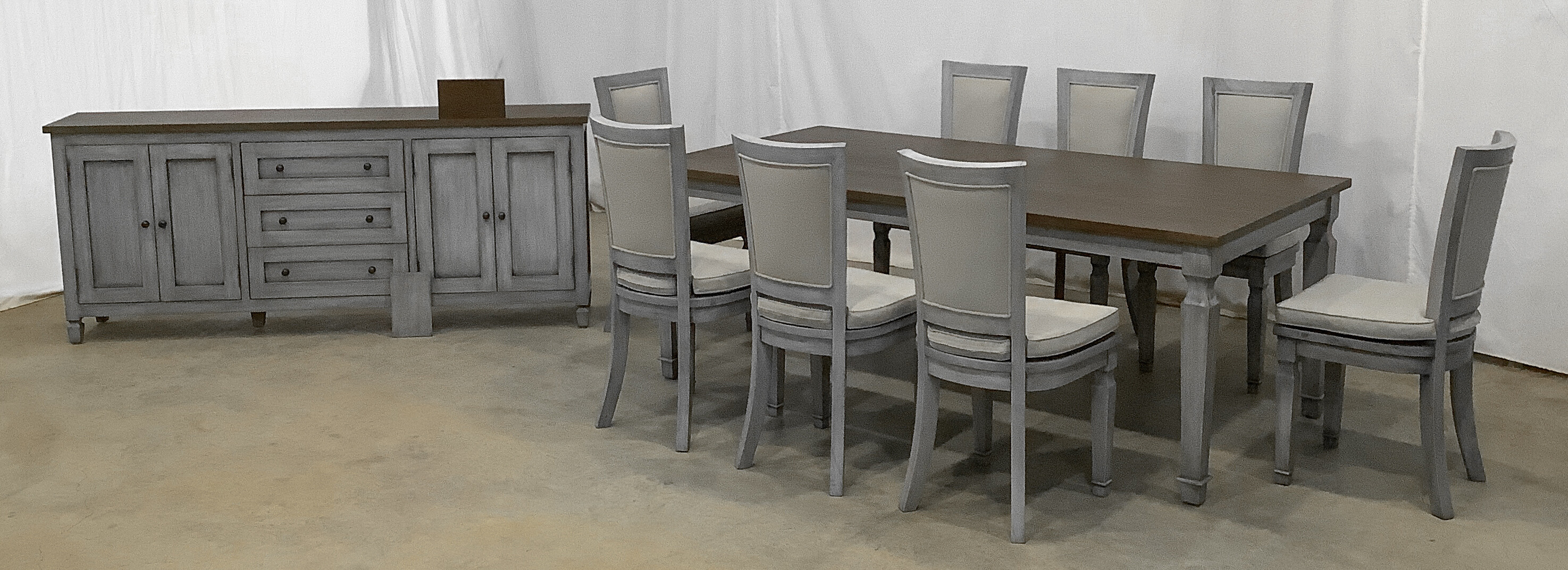In the image, there is a well-staged display of a dining room set within a furniture store showroom. The backdrop features a white panel accented by a curtain, creating a clean and inviting scene. The flooring below is a tan-colored concrete, adding a touch of modern industrial flair.

At the center of the display is a dining table with a dark brown wooden tabletop and gray legs. The table, exuding a sophisticated modern design, is paired with eight matching chairs—three along each of the longer sides and one at each end. The chairs share the same gray finish as the table's legs and frame, with additional features like light gray cushions and supportive backrests to enhance comfort.

Next to the dining table is a buffet server in a complementary gray color with a matching brown wooden top. This piece features two cupboard doors on each side and three central drawers, providing ample storage space. The consistent design elements and color scheme across the furniture pieces unify the display, making the set a visually appealing and cohesive ensemble for potential buyers.